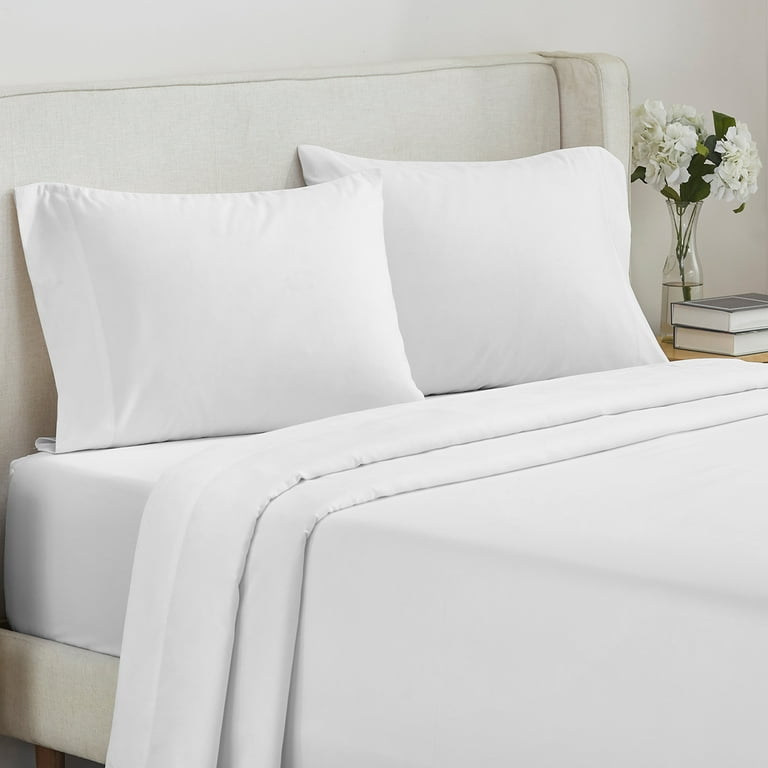The photograph is a square-format, color image capturing a neatly made queen or king-sized bed on a light gray fabric bed frame with an upholstered headboard. The bed is adorned with solid white bedding, including a fitted sheet and a comforter, which is partially folded over at the top. Two standard pillows in white pillowcases are propped against the headboard, facing outward. Beside the bed, on a light wood-colored side table, sit two large, black hardcover books stacked on top of each other. Additionally, a cylindrical vase, half-filled with clear water, stands on the table. The vase contains a floral arrangement of multiple white flowers and dark green leaves. The overall style of the photograph leans towards photographic realism and product photography, viewed from a slight angle from the headboard down to midway along the mattress.